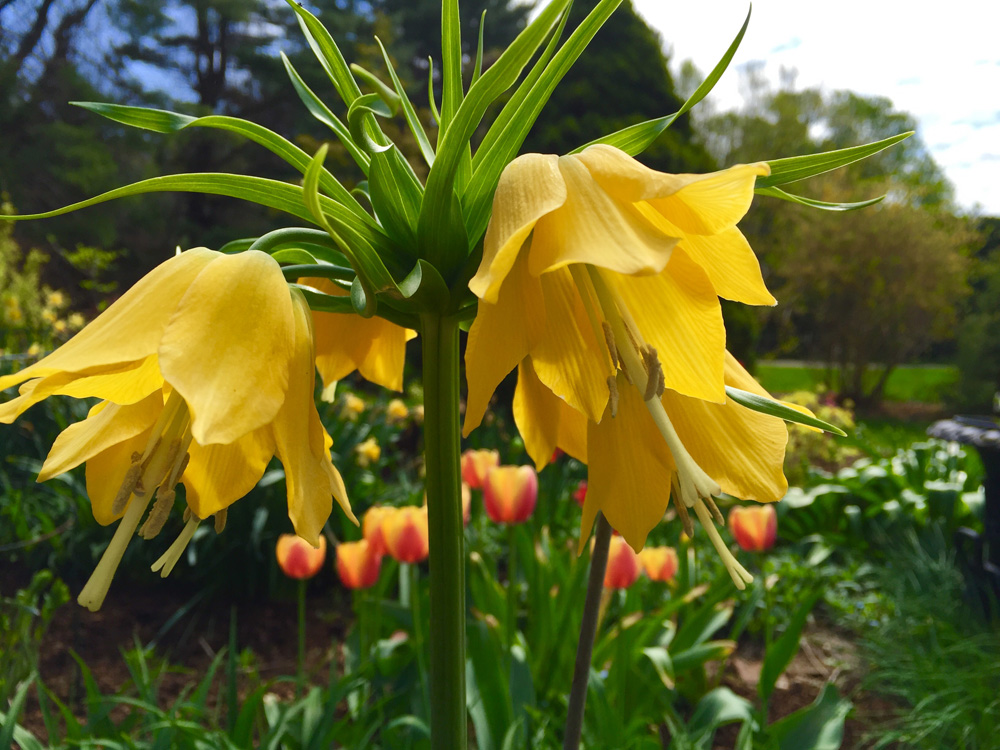This rectangular image showcases a close-up of a beautiful yet somewhat wilting flowering plant, possibly a tulip variety. Emanating from a thick, green stalk are two or three yellow flowers, each adorned with multi-petaled, almond or teardrop-shaped blossoms that are beginning to point downward. In the background, a row of vibrant yellow and pink tulips stands with their healthy green leaves, adding a lively contrast. The ground is a lush green carpet, leading up to a line of fully green trees that frame the scenery. The sky above transitions from a clear blue in the upper left corner to a subtly white hue in the upper right, encapsulating a picturesque springtime setting.